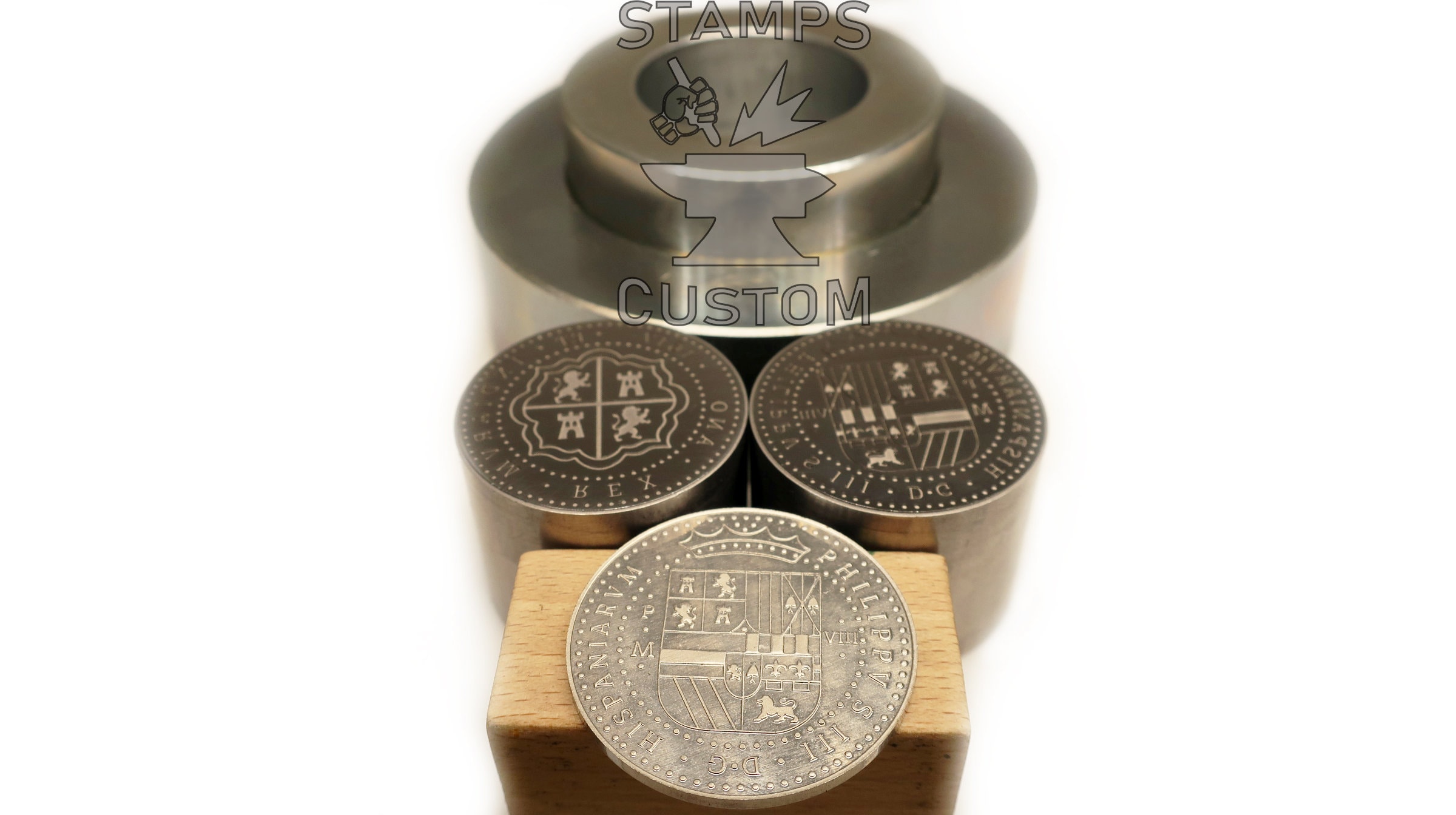The image showcases a promotional photo for custom metal stamps. Centered in a white background, a collection of intricately designed copper-colored items is displayed. The foreground features a cylindrical object that resembles a coin resting on a small wooden block. This coin bears the inscription "DC BEX OMA" and aligns with the designs on the other displayed equipment. Behind the coin, there are two similarly crafted smaller cylinders, apparently fitting into a larger hollow cylinder above them. The image suggests that the larger cylinder houses the smaller ones, potentially for stamping purposes. Above this arrangement, a watermark with the logo "Stamps Custom" accompanied by an anvil icon can be seen, emphasizing the item's purpose. The logo element suggests a metal stamping process, possibly for imprinting designs or text onto other metal objects.